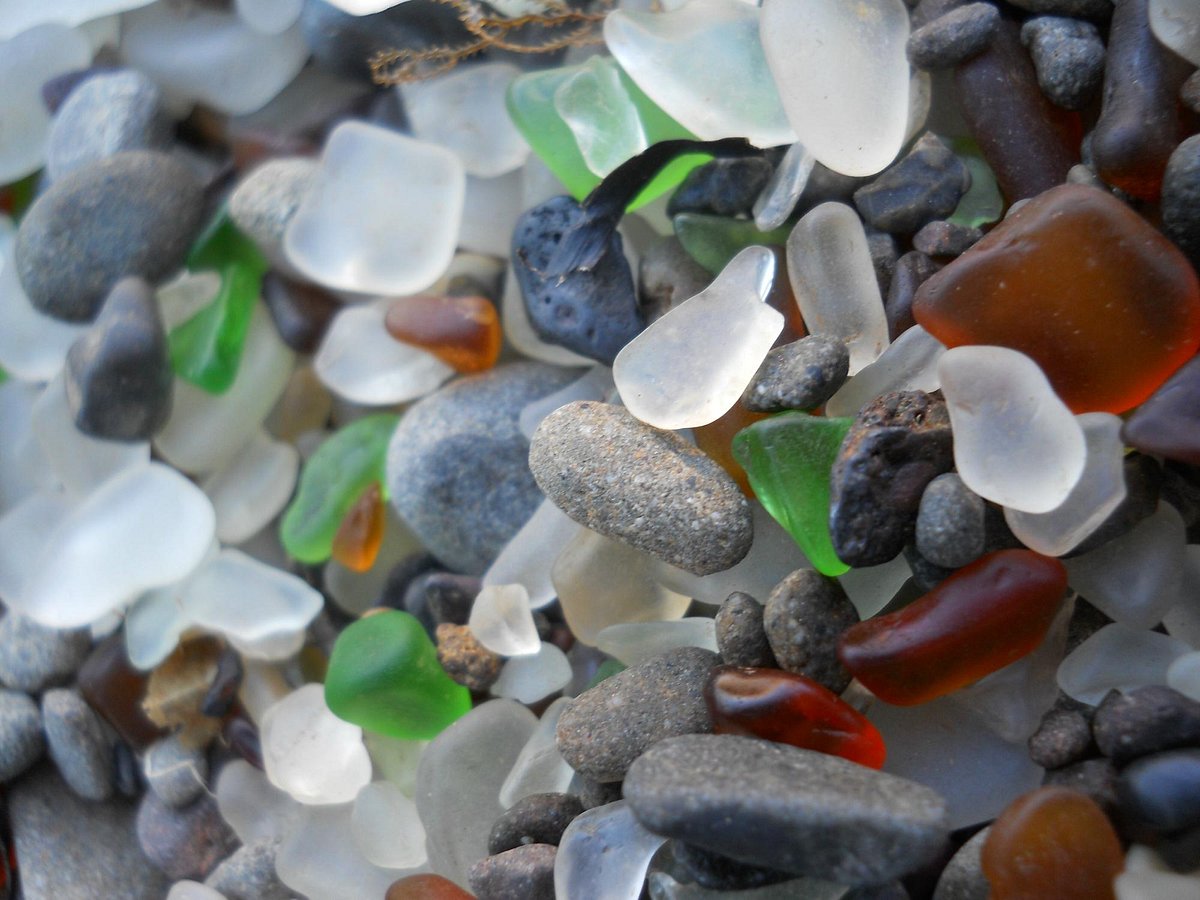The photograph showcases an extremely detailed close-up of a diverse mix of tiny, polished rocks and glass-like stones, resembling sand under high magnification. The array features a vivid palette of colors, including bright, translucent whites that resemble quartz, rich ruby rust reds akin to carnelian, deep greens reminiscent of jade or serpentine, and various neutral tones such as beige, tan, and gray river stones. Some stones have an almost glassy appearance with transparent qualities, while others display solid, opaque colors. Notably, there's a square orange stone and a perforated blue stone in the center. The scene is possibly set on a beach or riverbank, with hints of natural debris like plant material intermixed. The stones vary not only in color but also in size, ranging from tiny specks to slightly larger pebbles, all exceedingly smooth as though treated by a tumbler, giving the entire image a vibrant, mosaic-like quality.